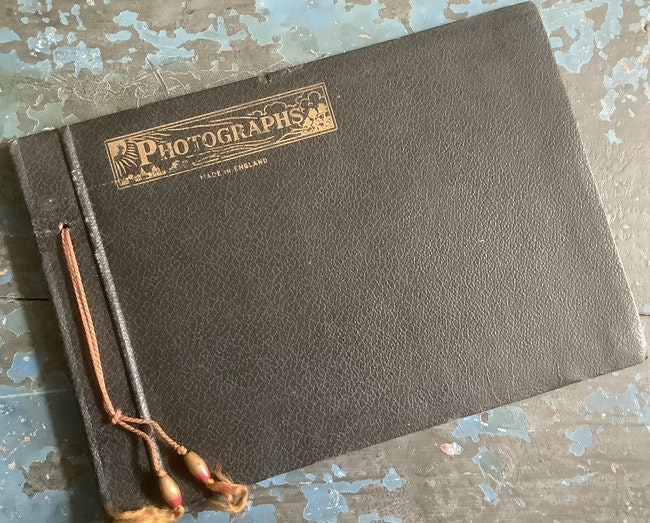The photograph reveals an aged, leather-bound photo album, distinguished by its elongated shape and classic design. The album's black leather cover is accented with a gold-stamped inscription in serif font, reading "PHOTOGRAPHS" in the top left corner. This inscription is housed within a tan bar, from which sunlight emanates, casting shadows of trees and a cluster of buildings across it. The book is angled such that its spine recedes to the bottom left, and partway down the spine, a small hole can be seen. From this hole, a yellow-gold or light brown string is threaded, wrapped around the album, ending in tassels shaped like vertical ovals. This photo album rests on a weathered surface with chipped gray paint intermingled with rusty blue speckles, adding to the vintage atmosphere.